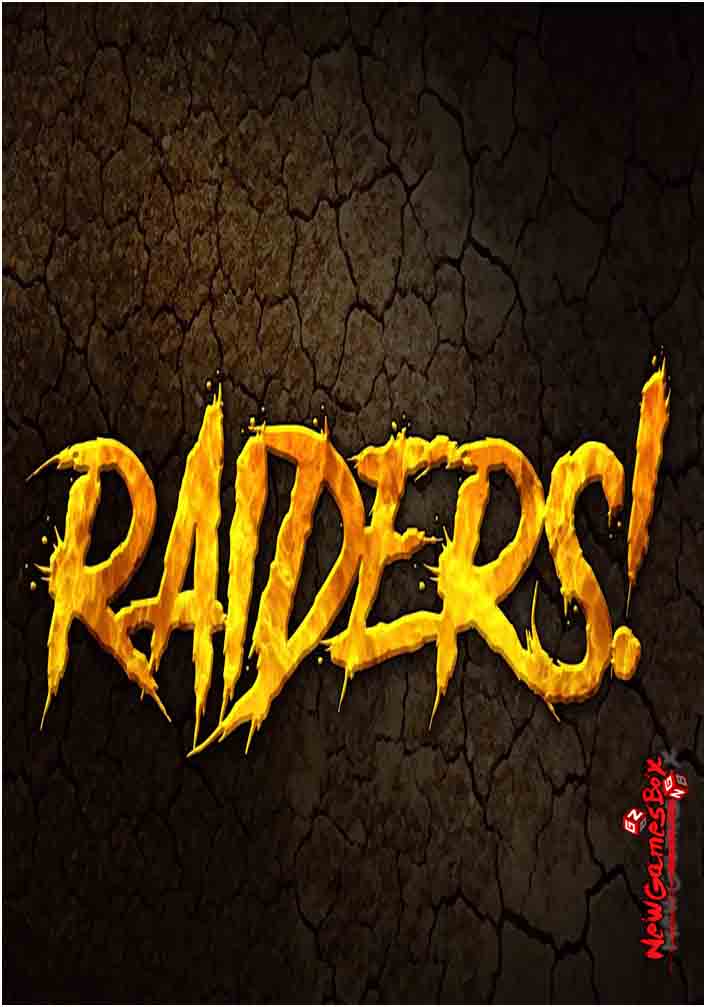The image from New Games Box appears to be part of a game-related material, possibly a title page, instructions, or an advertisement. It features a cracked, rocky, and dark brown background that resembles dried, muddy ground. Dominating the image is the text "Raiders!" in bold, capital letters. The font of "Raiders!" is goldish-yellow and styled to look wild with uneven letters and splashes, evoking a sense of flames or something rugged and intimidating. Additionally, in the bottom right corner, the text "New Games Box" is written vertically in red letters, starting from the bottom and moving upwards. Adjacent to this text are two dice, reinforcing the gaming theme.